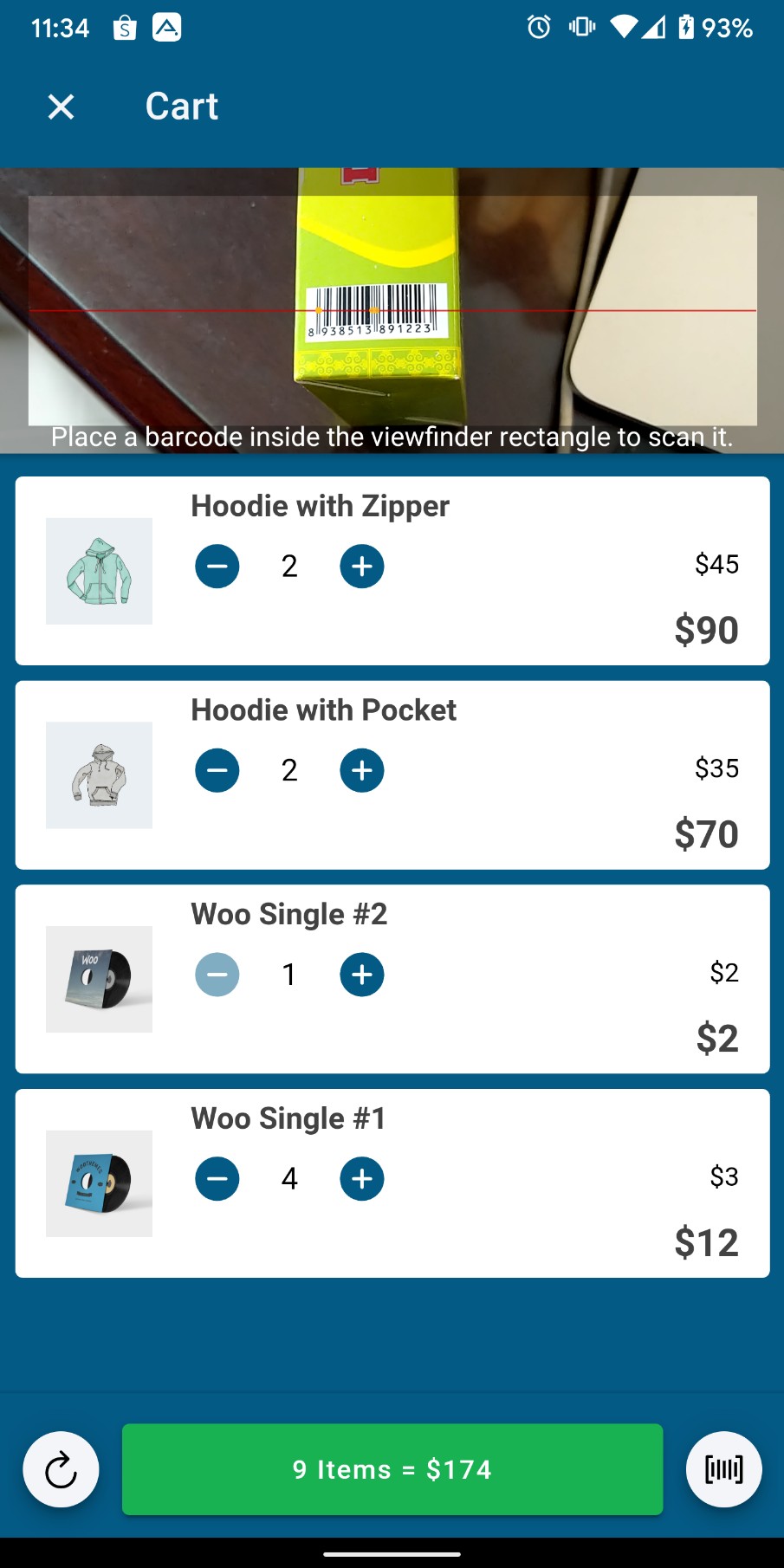This image appears to be a screenshot from a smartphone, displaying an e-commerce interface, likely from a shopping app such as Shopify. The top-left corner shows the time "11:34" with a row of app icons next to it, starting with the Shopify icon, followed by an unfamiliar square-shaped icon with an "A" in it, and then icons for a clock, toggle, Wi-Fi signal, a three-quarters full phone signal, and a battery indicator showing 93% in a blue banner. 

Below this banner, there is a closeable notification, indicated by an 'X' in a rectangular card to the right. Next, the main content shows a barcode scanner interface with a yellowish-green product on a table, labeled with a serial number. Text prompts the user to "place barcode inside the viewfinder rectangle to scan it."

Further down, there are four segmented sections displaying items for sale. The first section lists a "Hoodie or Zipper" with a product image, quantity controls (a minus sign, a number "2," and a plus sign), and the pricing information: "$45" per item and "$90" in total. Additional items displayed are labeled "Hoodie with Pocket," "Woo Signal Number Two," "Woo Signal Number One," each with respective media images and price listings on the right-hand side.

At the bottom of the screen, a green rectangle states "9 items equals $574," alongside a refresh button on the left and a barcode button within a circle on the right.